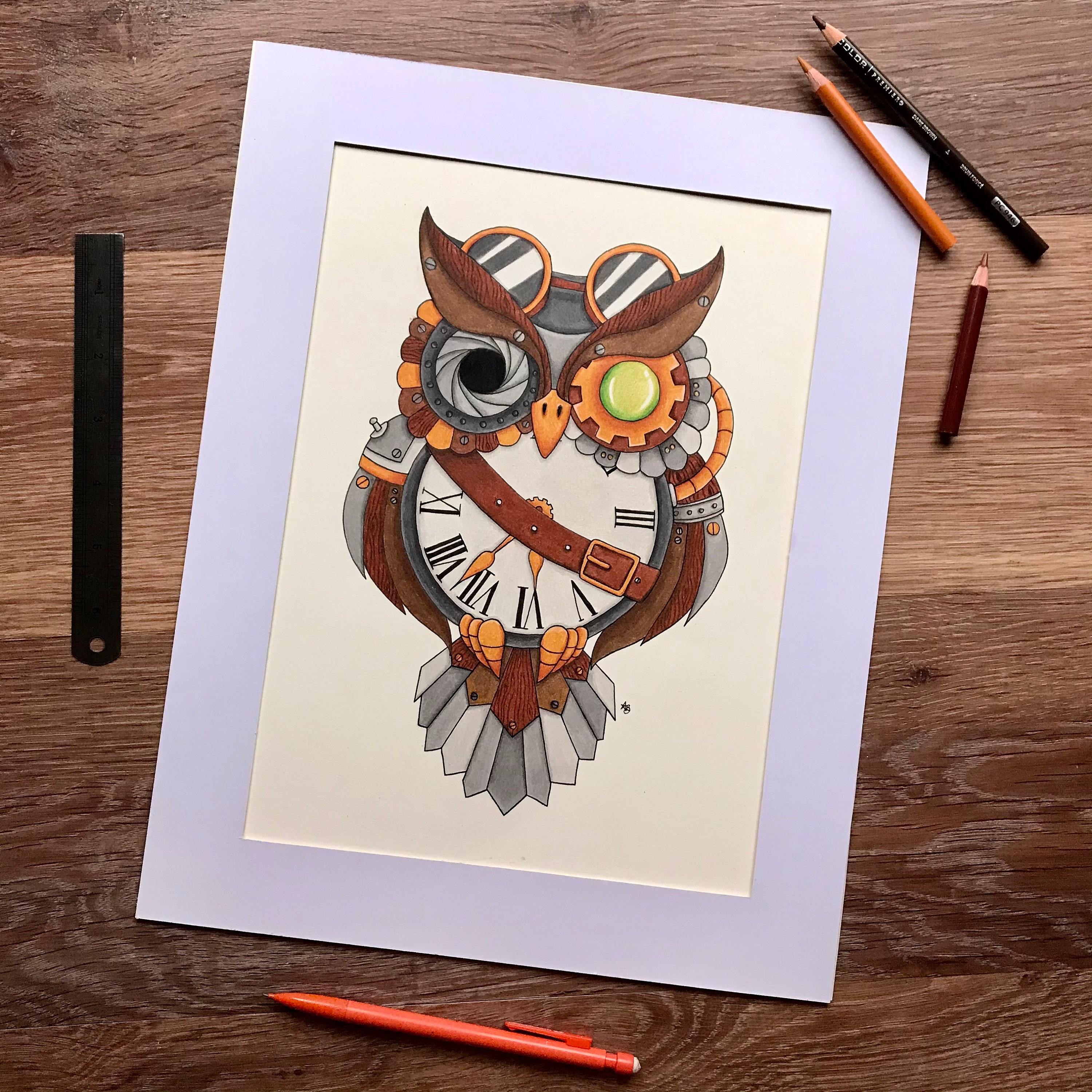This image displays a detailed drawing of a steampunk-inspired owl on a piece of white paper with a gray matted frame, all resting on a light tan wood surface accented by darker wood grain slats. The drawing is laid out diagonally from the bottom left to the top right. On the left side of the image, a black ruler, which has a hole at one end, stands vertically. Scattered around the drawing are colored pencils, including shades of black, brown, and orange, along with an orange mechanical pencil at the bottom. The owl, intricately designed with a clock face body featuring Roman numerals and clock hands, sports a leather strap with a goldish-brown buckle across its middle. It has two large, gear-like eyes and wears a set of goggles atop its head. Its wings and tail exhibit a combination of metal and wood elements, enhancing the steampunk aesthetic.